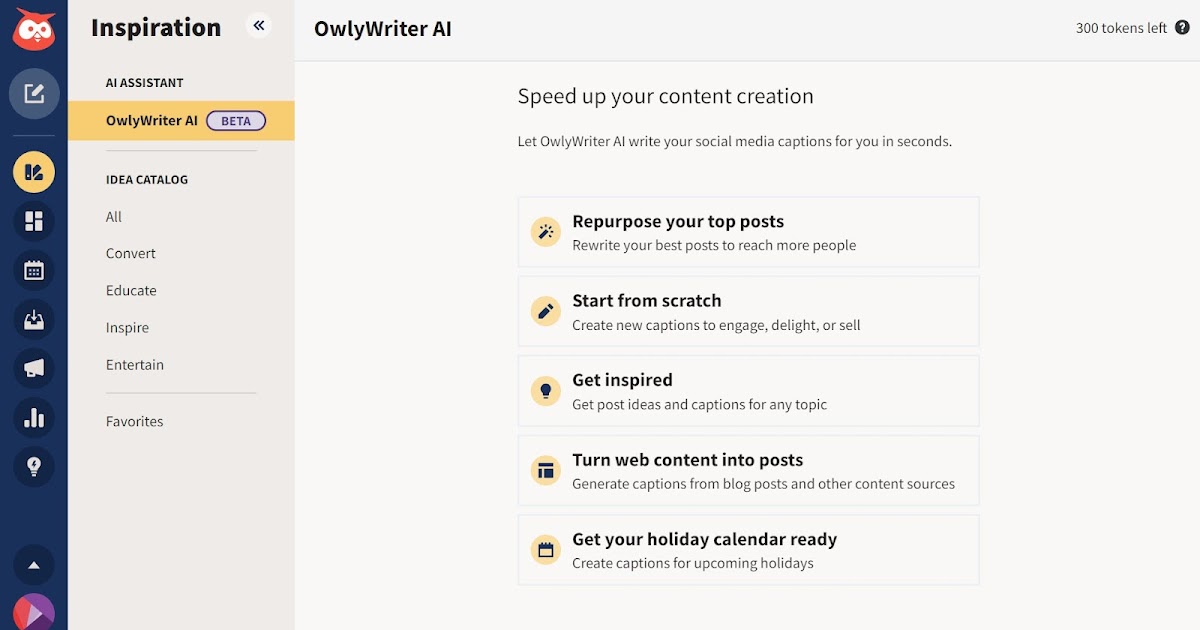The image features a sleek, grey background with prominent text and various icons. At the top, the text "AlleyRider AI - 300 tokens left" is displayed clearly. Below this, in a structured format, a series of engaging phrases outline the functionalities of AlleyRider AI:

- "Speed up your content creation," 
- "Let AlleyRider AI write your social media caption for you in seconds."
- "Repurpose your top posts," 
- "Rewrite your best posts to reach more people."
- "Start from scratch," 
- "Create new captions to engage, delight, or sell."
- "Get inspired," 
- "Get post ideas and captions for any topic."
- "Turn web content into posts," 
- "Generate captions for blog posts and other content sources."
- "Get your holiday calendar ready," 
- "Create captions for upcoming holidays."

Each statement is accompanied by a light brown circle icon that illustratively represents the corresponding action or feature. On the right side of the image, a sidebar displays categories in a list format including "Inspiration," "AI Assistant," "AlleyRider AI Beta," "Idea Catalog," "All," "Convert," "Educate," "Inspire," "Entertain," and "Favorites." This layout suggests a user-friendly interface designed to streamline social media management and content creation.